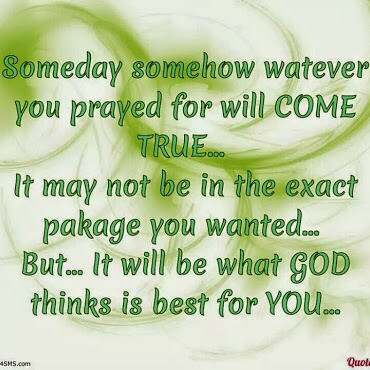The image features a predominantly text-based photograph with a backdrop composed of a white background interspersed with green areas that resemble rippling puddles. Dominating the center of the image is an inspirational quote written in dark green text: "Someday, somehow, whatever you prayed for will come true... It may not be in the exact package you wanted... but... it will be what God thinks is best for you." The quote spans across the entire screen. At the very bottom left, in small black font, there's a website link that appears to read "4sms.com." Additionally, the bottom right corner contains the word "Quote" in red text, though it is slightly cropped off. The overall aesthetic is simple yet evocative, with the green hue and ripples adding a serene touch to the motivational message.